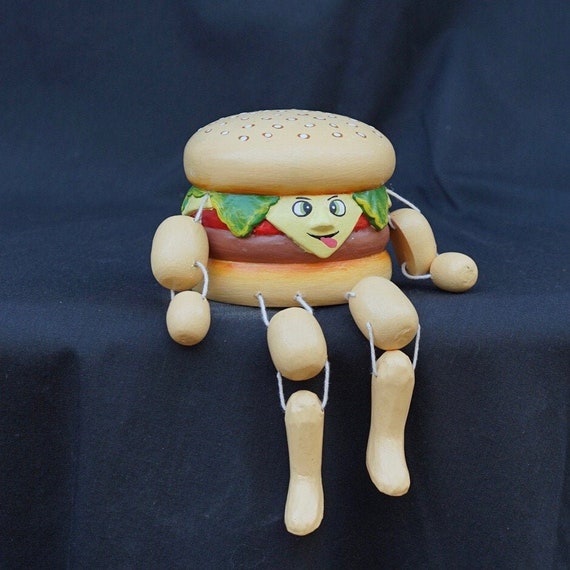Displayed against a black background in what appears to be a photography studio, the image showcases a whimsical figurine designed to resemble a cheeseburger with a human-like appearance. The cheeseburger features a face on a drooping triangular piece of cheese, complete with crossed eyes, a protruding tongue, and a small nose, giving it an endearing expression. The figurine mimics a 'shelf-sitter' or marionette with segmented limbs made from chiseled wooden pieces, attached by strings to resemble arms and legs. The cheeseburger includes all the classic components: a top bun sprinkled with sesame seeds, lettuce leaves peeking out, a juicy tomato slice, a hamburger patty, and the distinctive slice of cheese that forms the face. The figurine is placed on a ledge covered by a black cloth, emphasizing its playful, carved details and transforming the everyday burger into a charming, anthropomorphic character poised for display.